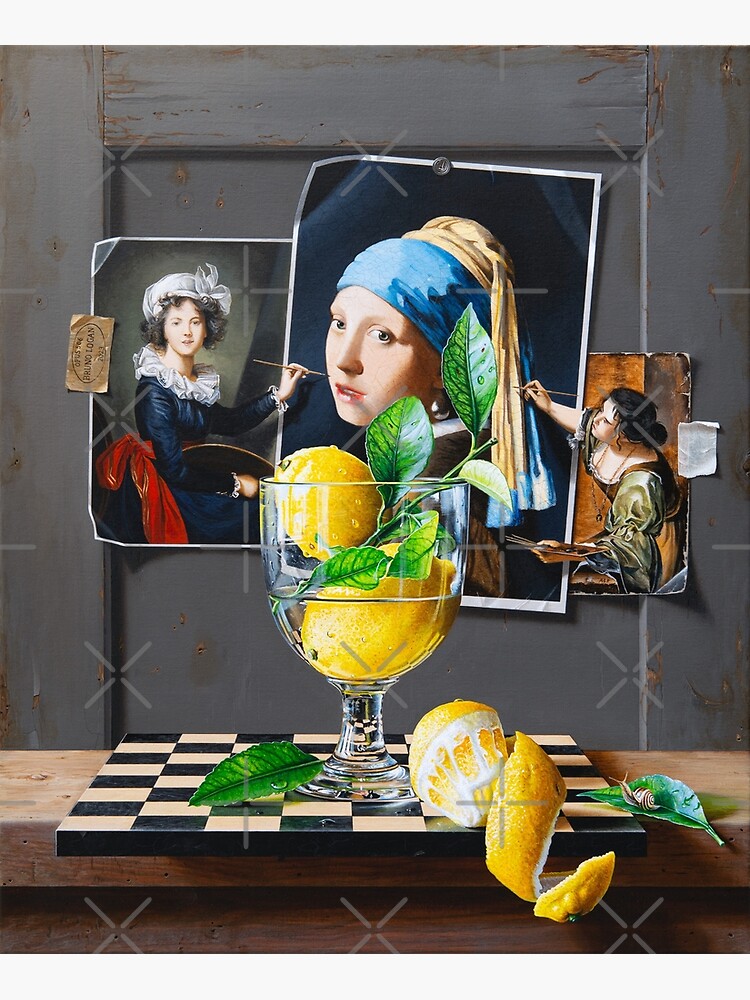This digital art piece masterfully fuses multiple classic paintings into a single cohesive composition. Set against a greyish painted wood panel background, the scene centers on a light brown wooden table, upon which a chessboard is prominently displayed. Atop the chessboard sits a partially spiralized lemon adorned with two mint leaves, accompanied by a small, detailed snail. Enhancing the enigmatic atmosphere is a clear glass goblet positioned on the chessboard, filled with water and holding additional whole lemons and mint leaves.

Dominating the background are three classical paintings. At the center is the iconic "Girl with a Pearl Earring," easily recognizable and rendered with blue and yellow hues in her headscarf, which may differ slightly from the original. Flanking this central masterpiece are two smaller paintings of women who intriguingly extend their reality by reaching out of their canvases. These women, one dressed in a blue dress with a red ribbon and a white hat, and the other in green attire, are actively painting the central artwork. Their paintbrushes and easels break the boundaries of their frames, creating a dynamic interaction between the paintings. These intricate details draw the viewer into a timeless blend of classical art and modern creativity.